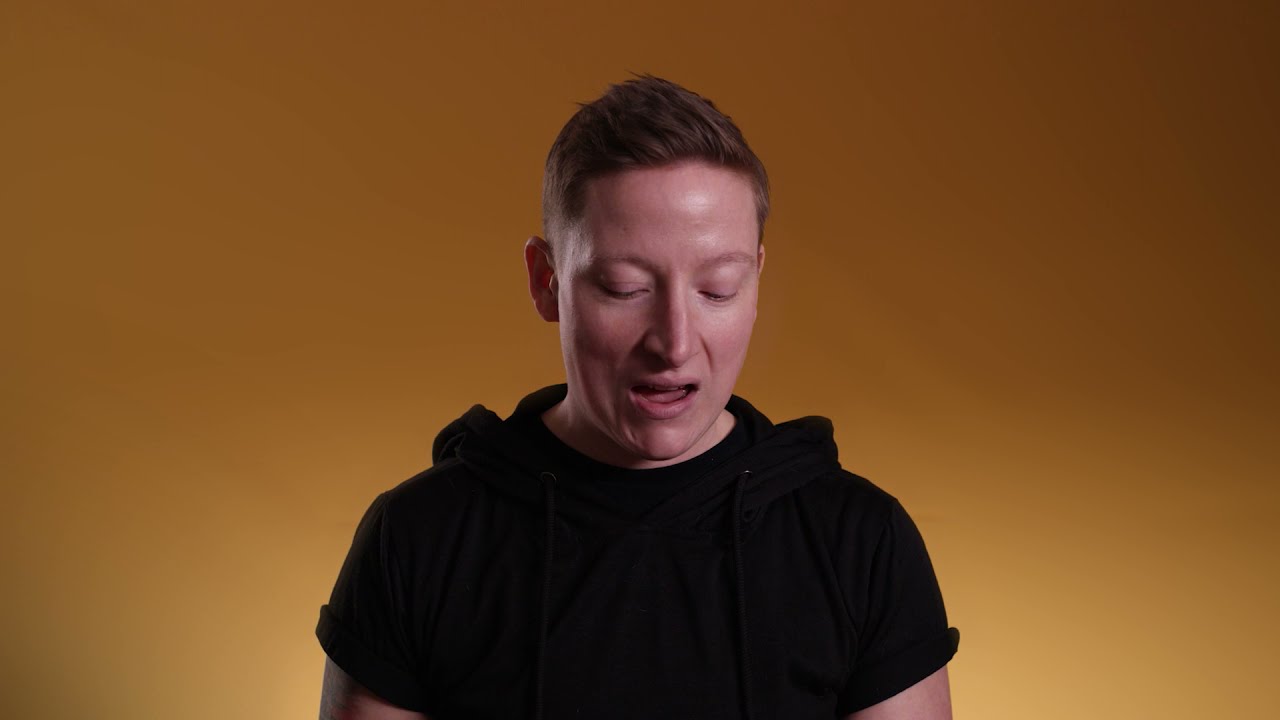The image features a white-skinned individual with short brown hair, sitting against a gradient yellow to brown background that darkens towards the top. The person is centrally positioned and is wearing a short-sleeved black shirt that resembles traditional monk attire, minus the hood. Their eyes are cast downward, and their mouth is open as if they are speaking, singing, or perhaps on the verge of sneezing. The image composition is minimal, with no additional objects or text present, highlighting the person as the sole subject in a scene that could be part of a TV show or YouTube video. The dominant colors in the image are black, yellow, and brown.